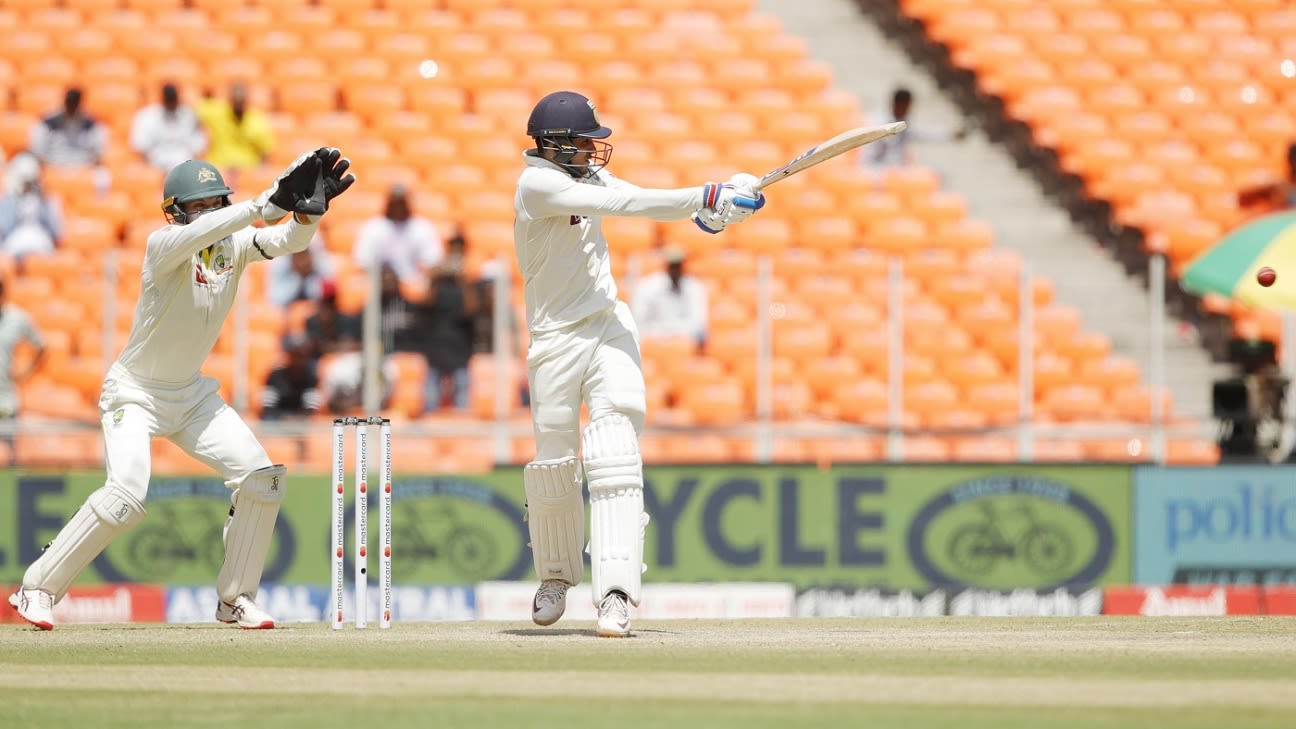The photograph captures an action-packed moment during a cricket game in a sparsely populated stadium. The backdrop features rows of orange seats, with only a few spectators dispersed among them. In the foreground, two players stand out on the green field, both donned in full white uniforms, including white shin pads and trainers. The batsman, wielding a white cricket bat, is mid-swing, having seemingly made contact with a red ball that is visible in the frame. He wears a dark blue helmet with a protective face cage. Positioned behind him is the wicket-keeper, poised to catch with his arms raised, wearing a light green helmet that suggests they're from opposing teams. Both players sport multicolored gloves. Advertisements line the lower walls of the stadium, with one promoting bicycles in green and blue letters, and another with blue text. A multicolored umbrella provides shade to a camera crew filming the game, adding to the vibrant and sunny atmosphere. The image, rich in detail, projects a dynamic and energetic scene, emblematic of a lively cricket match.